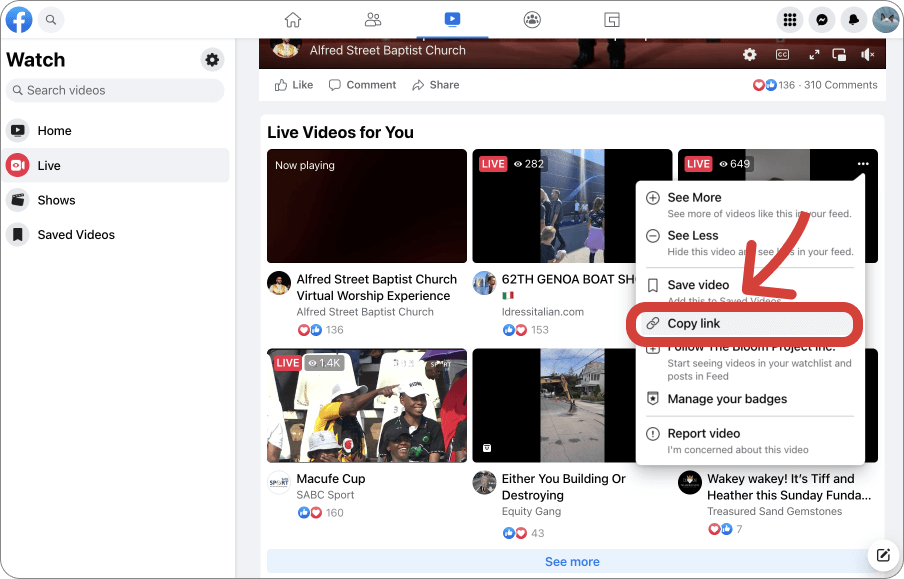Screenshot of the Facebook App Interface:

In this detailed screenshot of the Facebook app, the iconic Facebook logo is prominently displayed in the upper left-hand corner, adjacent to a search field. A series of navigational icons follows, including a home icon, a people icon, a video play icon, a friends icon, and a puzzle piece icon. On the right side of the top bar, there's a nine-grid square menu, a speech bubble menu, a bell icon for notifications, and a profile icon featuring a cat's face.

On the left-hand side of the screen, there's a vertical menu labeled "Watch" with a gear icon next to it for settings. Below this, options for "Search Videos," "Home," "Live," "Shows," and "Saved Videos" are listed. This menu is part of Facebook's video section, which might come as a surprise to some users.

To the right of this vertical menu is a horizontal separator, followed by a panel displaying videos in a format reminiscent of YouTube. At the top of this panel, a partially visible section indicates content from "Alfred Street Baptist Church," with options to "Like," "Comment," and "Share" these videos. 

Below, there is a section titled "Live Videos for You," arranged in a grid of three columns and two rows. In the upper right corner of this section, a drop-down menu can be accessed with options like "See More," "See Less," "Save Video," "Copy Link" (indicated with an arrow and highlighted with a capsule around it), "Follow," "Manage Your Badges," and "Report Video."

The currently playing video is from "Alfred Street Baptist Church," while other live videos display the number of viewers. Notable content includes a live video with a coffee cup icon, another suggesting that you are "either building or destroying," and a video in the lower right corner titled "Wiki Wiki, it's Tiff and Heather this Sunday, Fun Day."